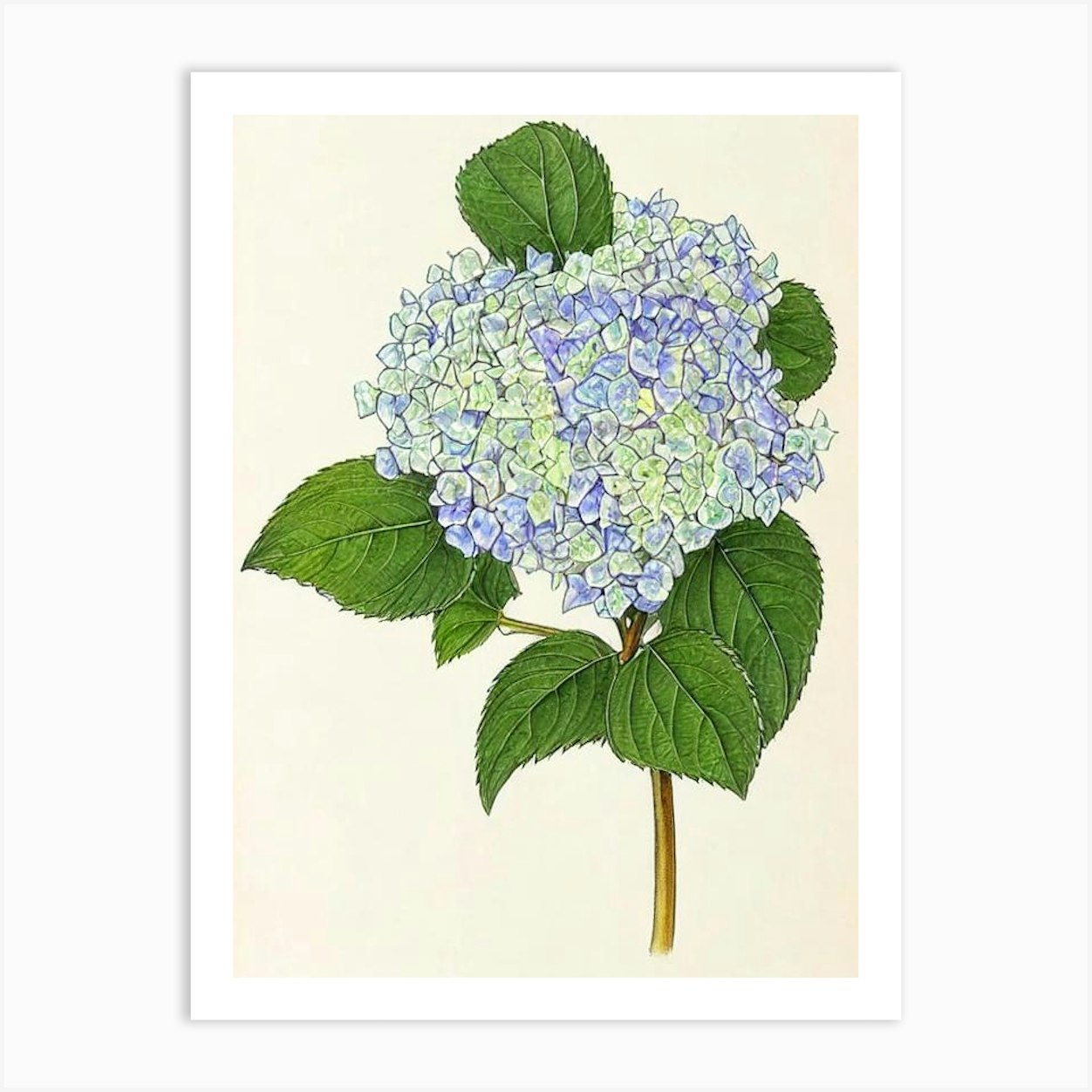This watercolor or colored pencil illustration, set against a crisp white square background with a pale gray wash, features a meticulously detailed depiction of a single hydrangea blossom, also known as a snowball bush. The hydrangea boasts a lush arrangement of approximately 100 individual flowers, predominantly in various stages of blue, lilac, and light green hues, capturing the dynamic transition from budding to full bloom. Some flowers exhibit a soft purple tint, enhancing the overall color diversity. The leaves of the hydrangea are strikingly green and prominently large, complementing the bloom with their lush verdure. Emerging from a slender, golden-brown stem, the vibrant flower heads and leaves seem to gently lean towards the left, adding a natural, dynamic movement to the composition.